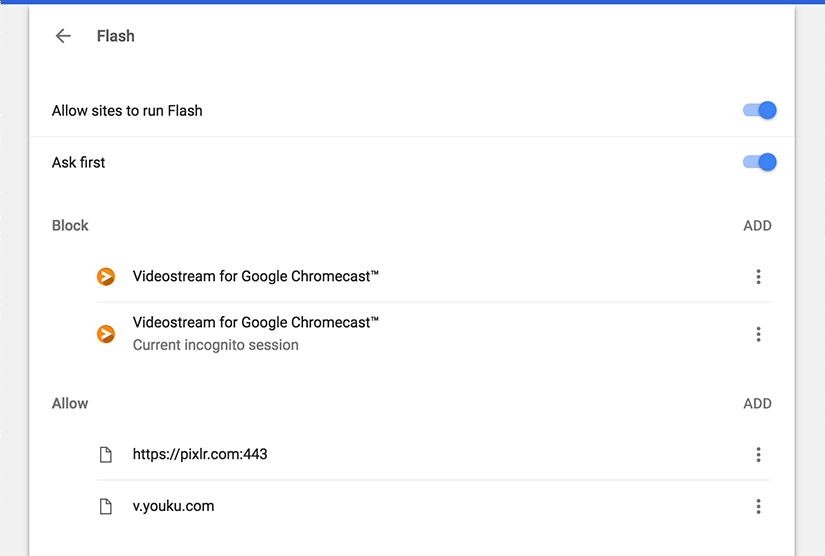The image appears to be a screenshot of a website interface for configuring Flash settings. The background is predominantly white with black text. In the upper left corner, there is a left-pointing arrow, and to its right, the word "Flash" is displayed, indicating this is the Flash settings menu.

Below the menu title, there is a section labeled "Allow sites to run Flash" accompanied by a bright blue slider that is toggled to the right, signifying that Flash is currently enabled. A gray horizontal line spans the screen, creating a partition.

The subsequent section is labeled "Ask first," with a similarly blue slider toggled to the right, indicating this setting is also active. Underneath, there is a section titled "Block," which seems to allow users to list specific sites where Flash is prohibited. Two entries under this section are "Video Stream for Google Chromecast" and "Video Stream for Google Chromecast Incognito, Current Incognito Session," both denoting blocked sites with respect to Flash. To the right of these entries is the word "ADD" in all caps, suggesting that users can add more sites to the block list.

Finally, there is an "Allow" section, which lists the sites permitted to run Flash. This section also includes an option to add new sites to the allowed list.